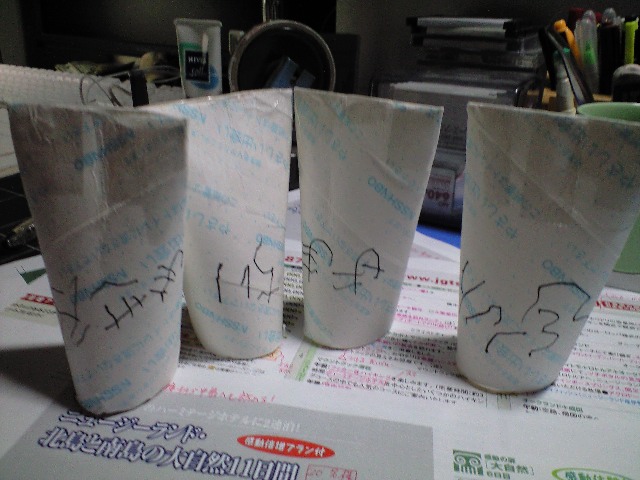In this low-light photograph, four cylindrical, white containers are prominently featured on a white table. Each container, resembling widened tubes of toothpaste or paper rolls, is round at the bottom and pinched shut at the top with tape. The bottom halves of these containers are adorned with oriental writing in black pen, while additional diagonal and pale turquoise blue writing also decorates the surfaces. The containers appear to be placed on a large paper or poster bearing more oriental writing, possibly a menu. The background looks cluttered and dimly lit, revealing what seems to be office supplies like pens, markers, and a cup, giving the impression that the setting could be an office or a home workspace.